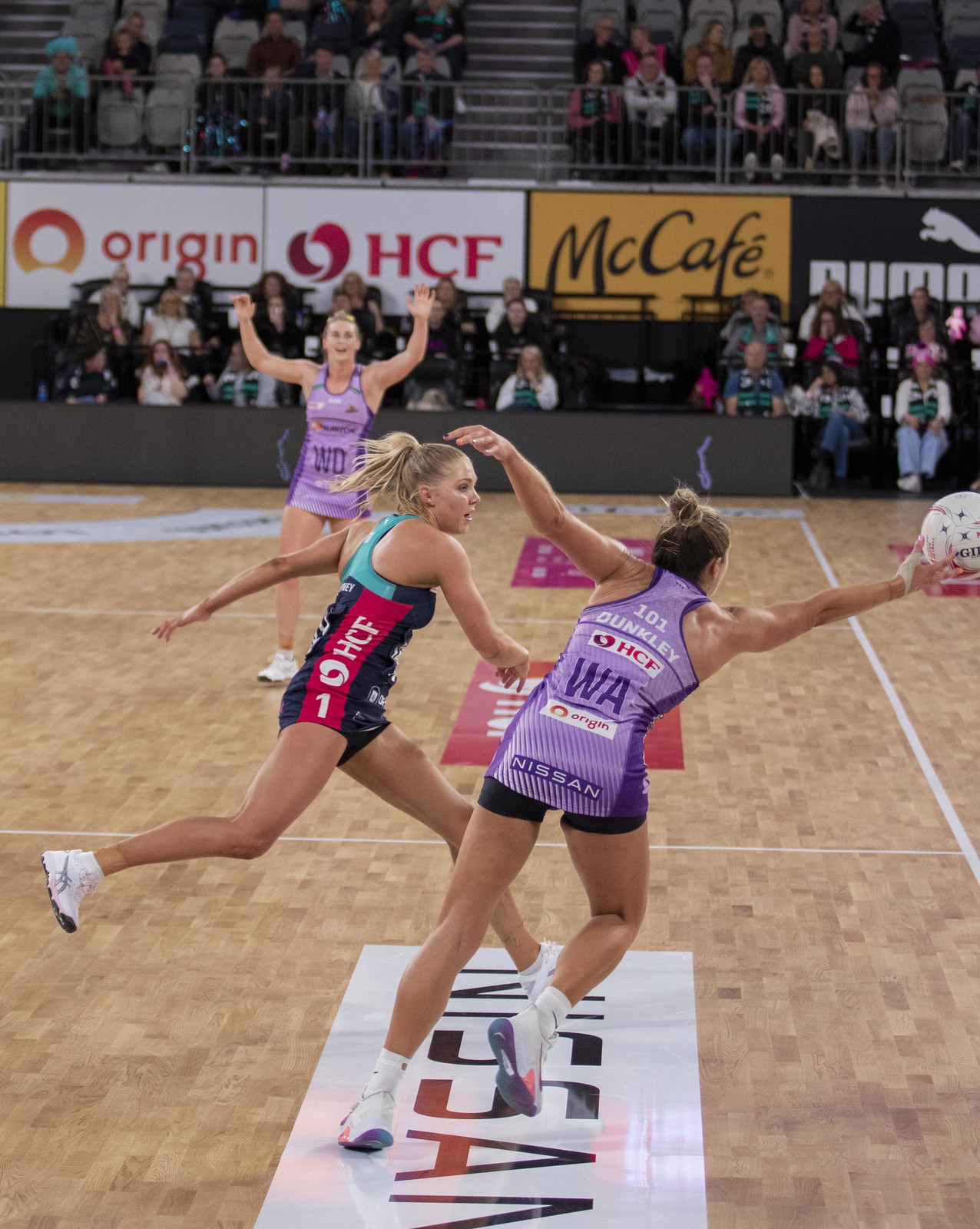The image captures an intense moment in a girls' high school volleyball game, taking place in an interior auditorium with polished wooden floors marked with white lines. The game is set in a relatively intimate atmosphere, with spectators visible in the background sitting in the stands. Prominent sponsor labels, including Origin, HCF, McAfee, and Puma, are displayed around the court, adding a splash of commercial color to the scene.

In the foreground, two athletic women are in dynamic action. One of them, wearing a purple jersey with the initials "WA," presumably representing Washington, is reaching out for a volleyball. Her hair is tied back in a bun. Her jersey features sponsors HCF, Origin, and Nissan. Beside her, another player in a striking light blue and dark blue jersey with a red stripe is rushing over to intercept the ball. This player, easily identified by her blonde hair pulled back in a ponytail, showcases the opposing team's colors.

Additionally, another purple-jerseyed player is visible in the background with her hands raised, ready to receive the ball. Together, the scene narrates a moment of strategic play in a closely contested volleyball match, amid the supportive but modest crowd.